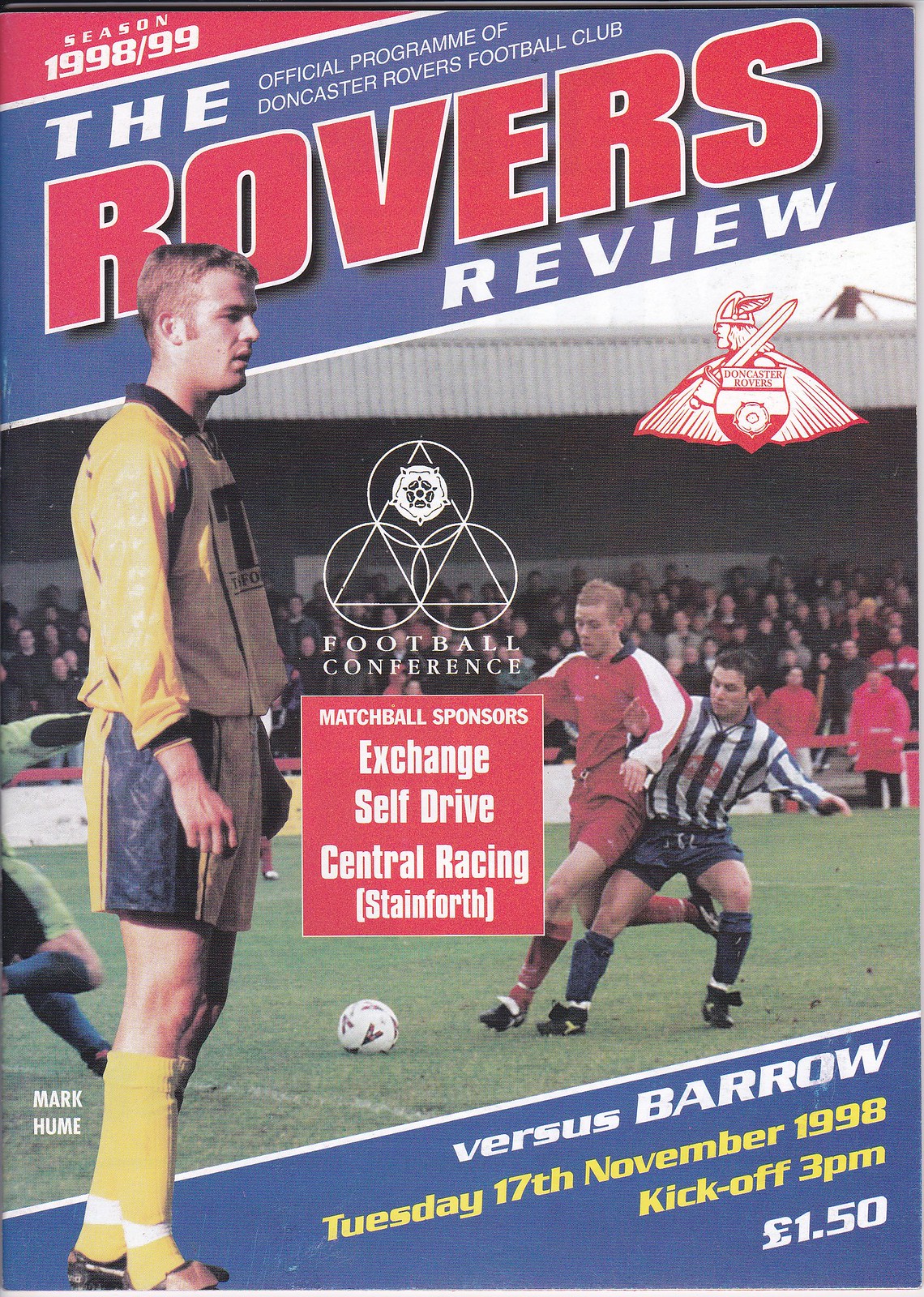The image is the cover of a soccer program, prominently featuring action on a vibrant green field. In the foreground, two players are vying for the ball: one in a red jersey, red shorts, and red socks, and another in a black-and-white striped uniform. To the right, a player in a yellow jersey with a black collar, yellow shorts with black sides, and yellow socks with white stripes is standing, looking right. Superimposed on the page is a large image of Mark Hume, also in yellow. The cover, from the 1998-99 season, displays "Rovers Review" in large red and white letters against a blue background. Below it, the program details the match: Doncaster Rovers versus Barrow, Tuesday, 17th November 1998, kickoff at 3 p.m., priced at £1.50.